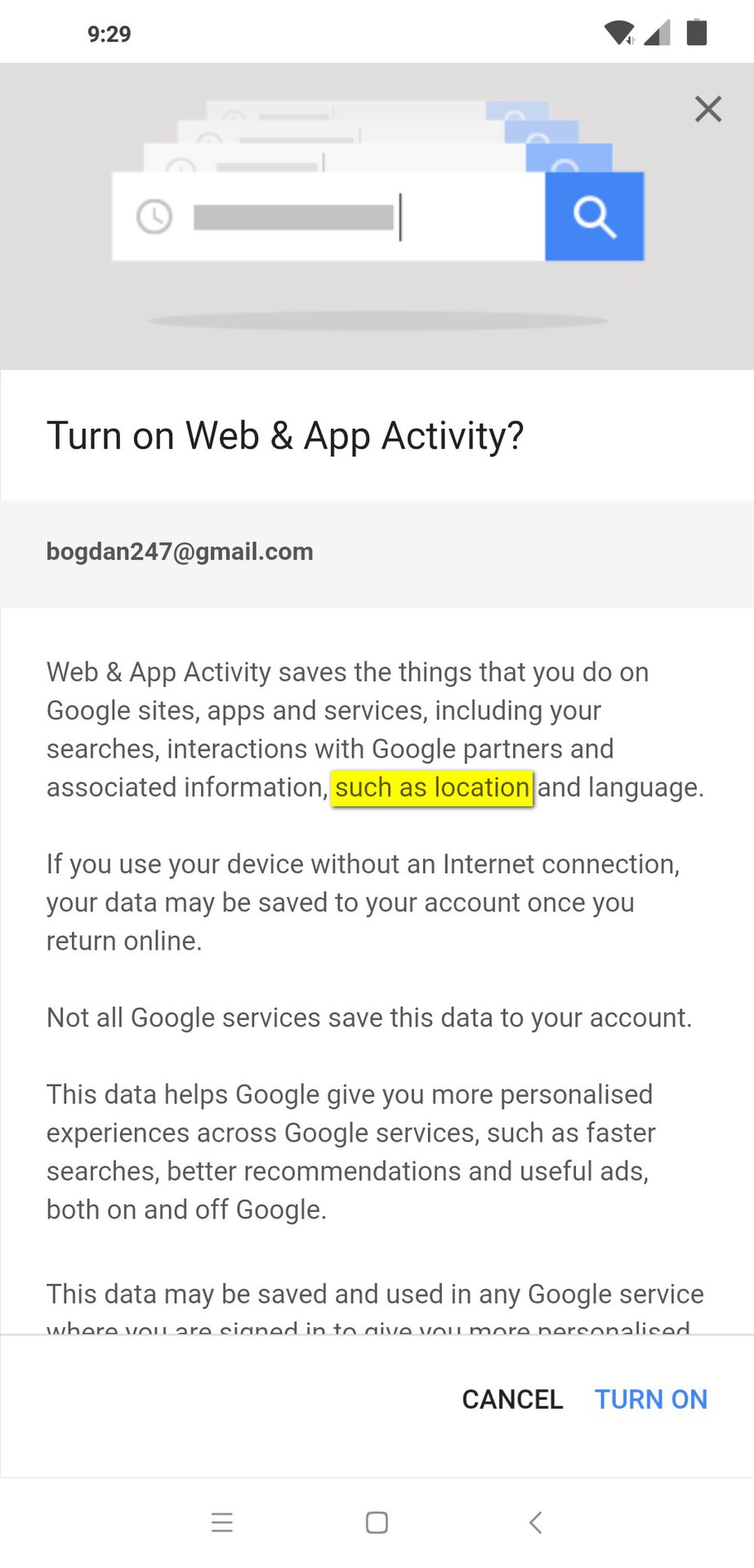### Detailed Caption:

The image appears to be a screenshot from a user's browser, specifically showcasing a Google account-related page, possibly within the Chrome or Gmail settings. At the top, there's a browser navigational bar characterized by a minimalistic design, featuring a clock icon, a search box, and a blue magnifying glass icon.

Prominently displayed is Google’s prompt to "Turn on Web and App Activity," indicating that this setting is currently disabled or awaiting user action. Beneath this prompt, the email address "bogdan247@gmail.com" is visible, identifying the logged-in user.

The main content of the page elaborates on the "Web and App Activity" feature. It explains that this feature tracks and saves user interactions across Google sites, apps, and services, including searches and interactions with Google partners. The text specifies that this collected data may include items such as location and language, with "location and language" highlighted in yellow. This highlighting draws attention to these specific data components, emphasizing their importance in personalized services.

Further details state that if the user operates their device offline, the data will be saved to their account once the device reconnects to the internet. It clarifies that not all Google services store this data in the user’s account. The purpose of saving this data is to enhance user experiences across Google services through faster searches, better recommendations, and tailored advertisements, both on Google’s platforms and elsewhere. The explanation cuts off mid-sentence, hinting at more benefits and uses of the data.

At the bottom of the screenshot, two buttons are visible: "Cancel" and "Turn on," offering the user a choice to either decline or enable the Web and App Activity tracking.

The overall color scheme of the page is muted with shades of gray, black, and minimal pops of color, contributing to a streamlined and professional interface design.